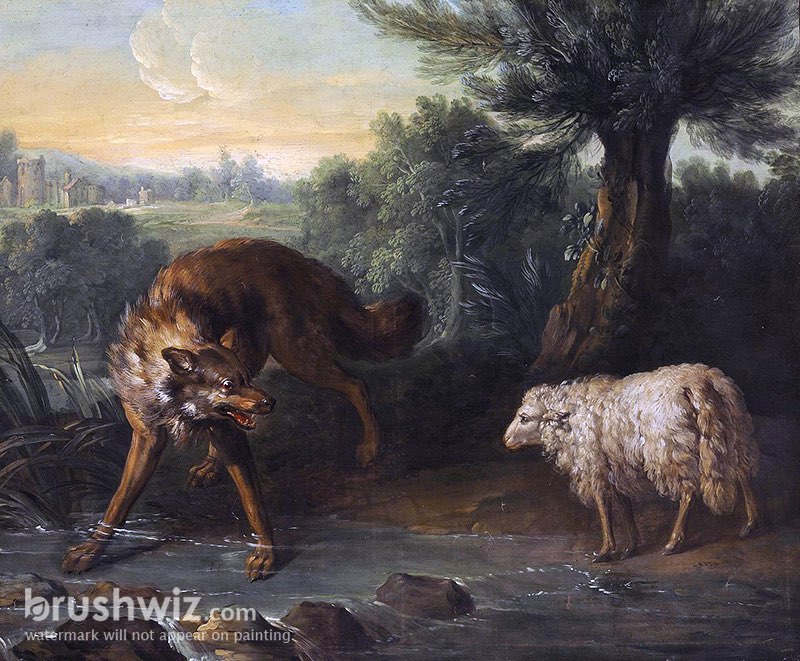This detailed painting, reminiscent of an older style oil painting, depicts a tense moment between a wolf and a sheep set in a naturalistic landscape. The wolf, standing to the left with a brownish coat highlighted by lighter patches, has its front legs splayed wide in a shallow, clear stream bordered by rocks. Its mouth is open, baring teeth in a menacing snarl, with wide eyes fixed on the sheep. The sheep, fluffy and predominantly white with some brown dirt stains, stands placidly on the right, seemingly unperturbed by the wolf’s threatening stance. The stream, which trickles gently through the scene, has a dark grey hue with visible rocks and a dark bank behind it.

In the background, a large tree with expansive foliage spreads outwards, partially obscuring a castle-like house set against a backdrop of fluffy clouds and a gradient sky tinged with blues and yellows, suggesting either sunrise or sunset. The setting is enriched with dark green bushes and extends into a dense forest, with foliage painting an earthy tone canvas. A watermark reading "brushwiz.com" is positioned in the lower left corner, noting that it will not appear on the final painting. This piece combines impressionistic elements with classic and earthy color tones, rendering a vivid and dramatic snapshot of nature.